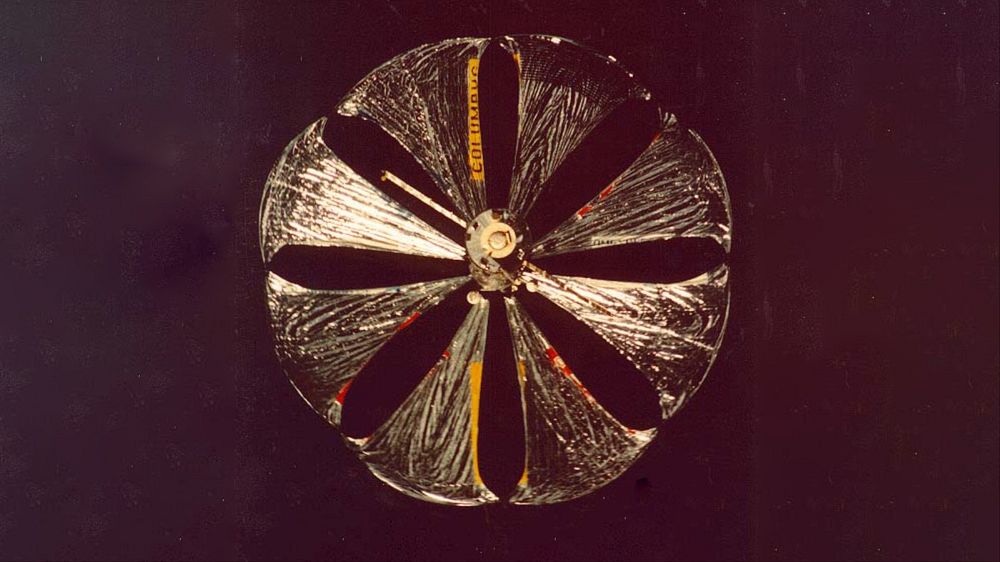The photograph depicts a top-down view of an intriguing object that resembles both a wheel and a parachute. At the center of the image, there is a cylindrical metal structure with a small hatch at the top. Radiating from this central metal piece are eight translucent, horn-shaped projections, which might be made of plastic or glass. These projections fan outwards like the petals of a flower or the canopy of a parachute that's in mid-descent, with gaps between each one. The entire assembly is set against a mottled dark brown background tinged with hints of gray and red. Notably, one of the translucent projections bears a label with an orange background and black lettering that reads "Columbus." Additionally, there are small bits of red and yellow print on the projections, adding to the intricate details of the object. The overall composition is reminiscent of a shuttle's parachute seen from above as it prepares for splashdown, blending both mechanical and organic elements in its design.